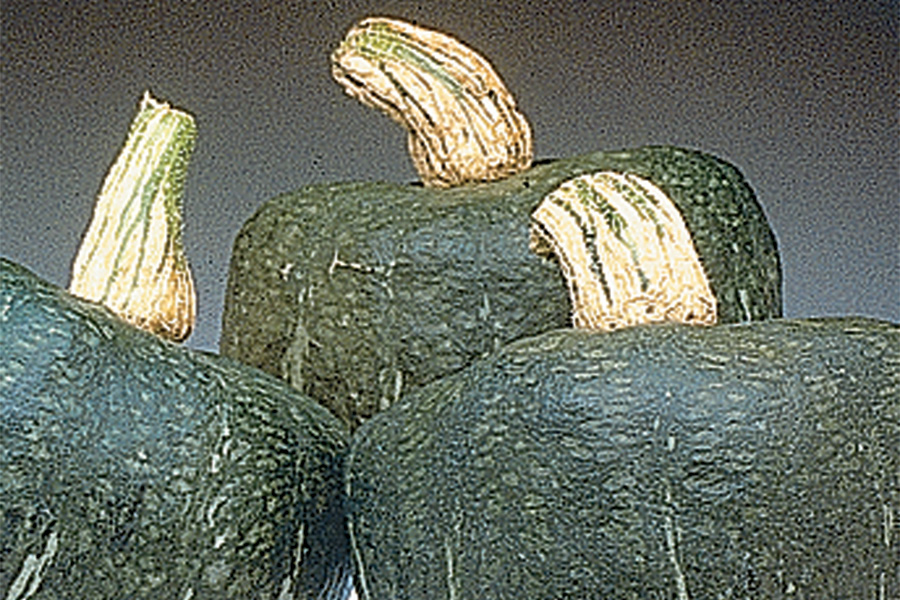This image, likely a photograph but possibly a painting, depicts three dark green squash resembling oversized green peppers. Their unusual shape diverges from typical squash or pumpkin contours, instead almost appearing like massive peppers. The squash feature a spackling of white or lighter green dots and specks scattered across their surfaces. Each of the three squash is adorned with a thick, textured stem demonstrating a mix of white and green hues. These stems are remarkably prominent, reminiscent of dried umbilical cords, and curve in different directions: the back stem curves left, the front right stem curves towards it, and the left stem stands straight.

The arrangement of the squash forms a sort of pyramid, with two at the base and one atop. The dark, almost black olive-green skin is marked by scratches and blemishes, hinting at a life spent growing under the sun or some rough handling. The background is a fuzzy gray fading into black, adding to the image's grainy, night-vision-like quality. Despite the overall low resolution and static-laden appearance, the details of the textured stems and marred surface of the squash stand out prominently.